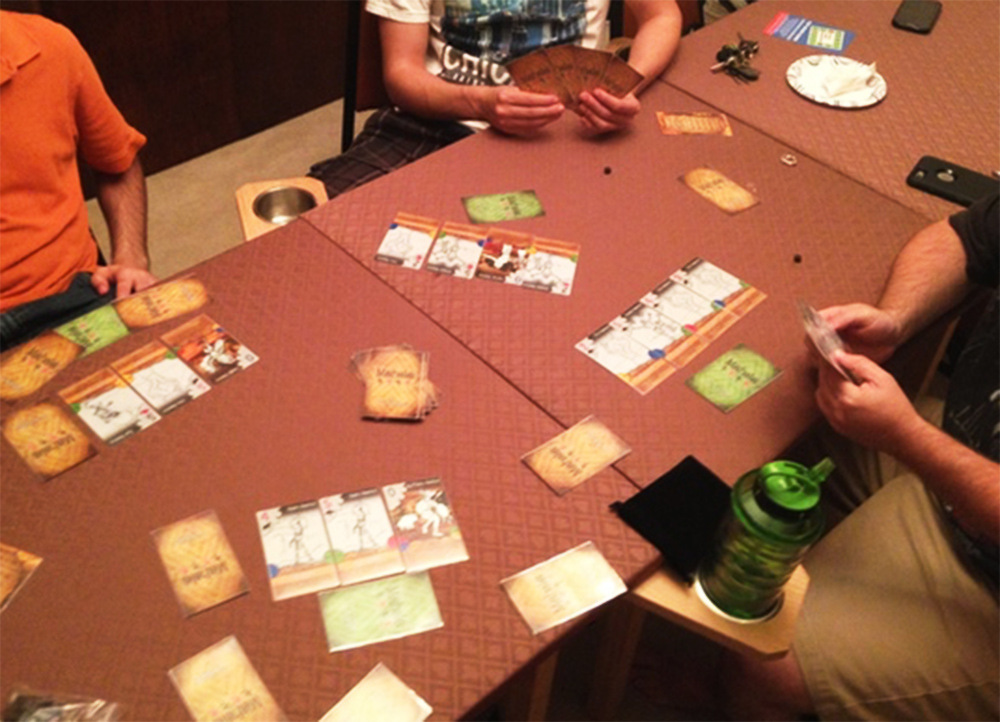In this engaging scene, three individuals are immersed in a card game. They are seated around a makeshift square table formed by pushing three red tables together. The layout begins from about halfway up on the left side, slanting up to approximately two inches from the right corner, and extends downward, just left of the center, connecting back to the middle on the right side.

The table surface is scattered with various cards, including some with brown backs, some green, and others turned face-up displaying cartoon characters. To the upper right, a white plate can be observed along with keys to its left, a phone positioned below the keys, and another phone situated in the upper right corner of the table.

Focusing on the individuals, the person in the top left corner is partly visible. He wears an orange short-sleeve shirt and blue jeans. His left hand rests on his thigh, but his head is out of the shot. Additionally, the setting reveals a section of the brown floor and a dark brown wall in the background.

Beside him, up from his position, another person appears. This individual is clad in a white short-sleeve shirt that features an illustration of a city. He wears dark black pajama pants and is holding three cards with brown backs.

In the bottom right corner, only the arms of the third player are visible, extending outwards to the left while holding cards. He is dressed in a black short-sleeve shirt and khaki pants. Nearby, to the left under the table, a brown drink coaster supports a green canister.

This detailed snapshot captures the lively essence and intriguing details of a casual yet captivating card game among friends.